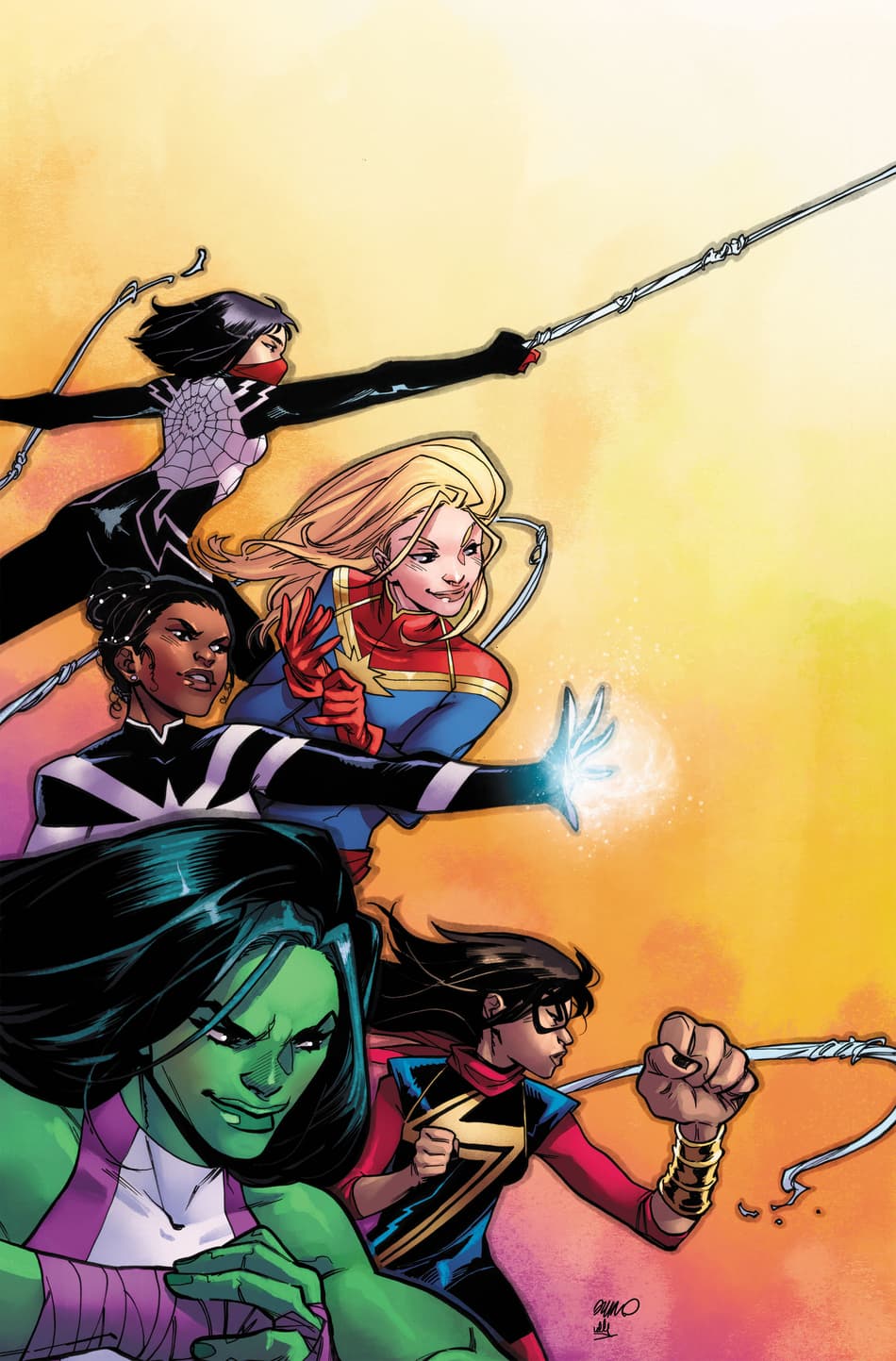The vibrant comic book-style illustration features five dynamic female superheroes, each poised strategically on the left side of the image against a gradient background that transitions from purple in the bottom left to white in the upper right. At the top, one superhero, distinguished by her dark hair, dons a black suit adorned with a purple spider web motif and a red face mask, brandishing a spear-like weapon. Just below her, to the right, a blonde-haired figure reminiscent of Superman or Captain Marvel tightens her red gloves, dressed in a striking red, yellow, and blue suit. Following her is an African American superhero in a black and purple-striped outfit, with her hair elegantly pulled back into a bun and a glowing hand stretched forward. Below, on the left, a powerful female resembling She-Hulk stands with green skin, black hair, and a purple and white uniform, confidently clenching her fist into her palm. Adjacent to her, slightly to the right, is a younger heroine in a red, black, and gold suit, adopting a fighting stance with one disproportionately large and elongated left arm, hinting at her ability to enlarge her fists. The composition concludes with a subtle black squiggle in the bottom right, likely the artist's signature.